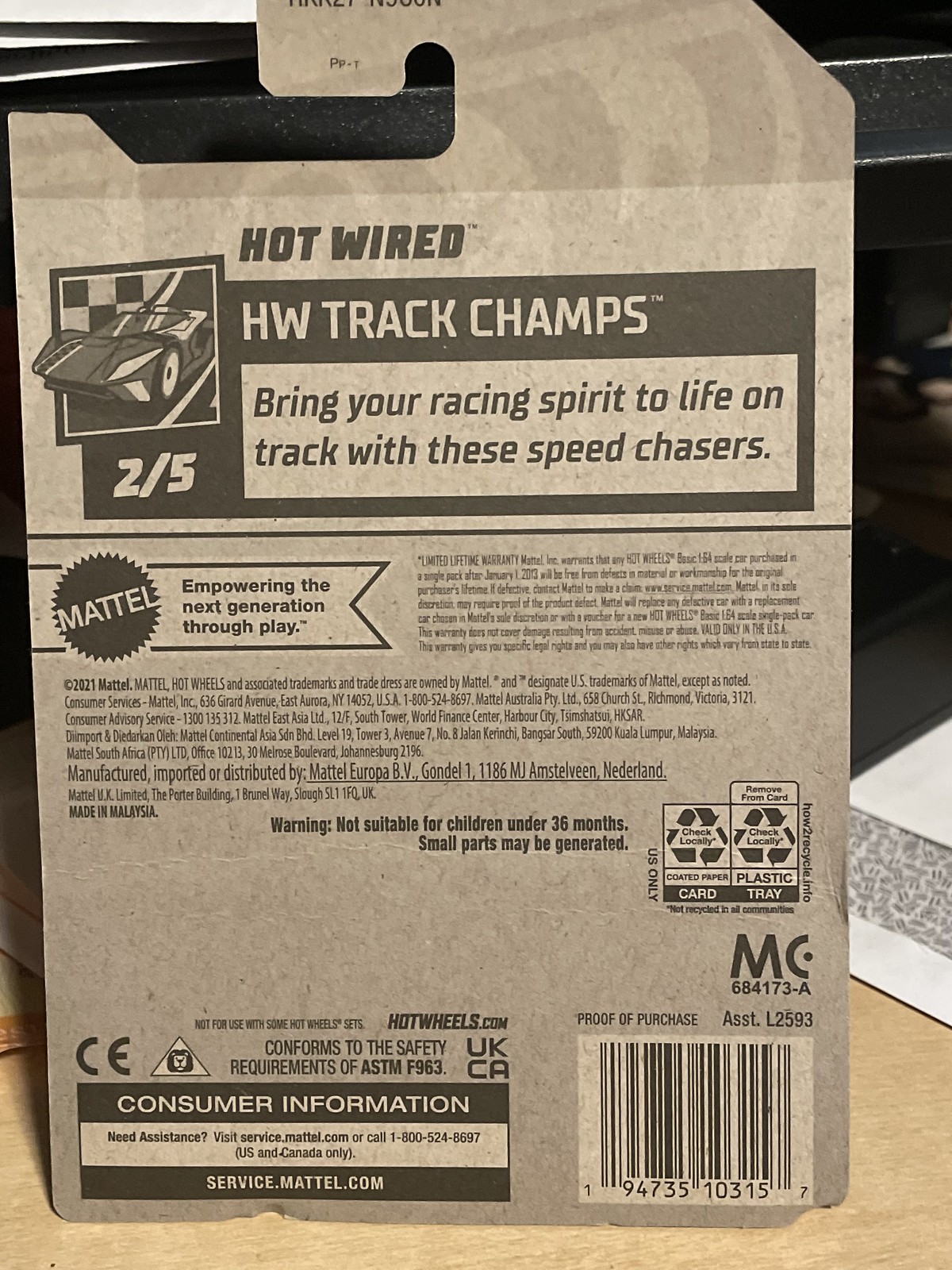The image features the back of a Hot Wheels toy packaging, specifically from the "Hot Wired HW Track Champs" series by Mattel, showcased on a grey cardboard background designed for hanging on store racks. At the top, in bold black lettering, it reads "Hot Wired HW Track Champs" and encourages consumers to "Bring your racing spirit to life on track with these speed chasers." Below this phrase, there's an illustration of a sports car, indicating that this is number 2 out of 5 in the series. The Mattel logo, a circle with multiple points around it, is prominently displayed with the tagline "Empowering the next generation through play." Additional fine print includes a limited lifetime warranty, copyright from 2021, warnings that the product is not suitable for children under 36 months due to small parts, and information about recycling the cardboard tray. There's a barcode at the bottom right and a consumer information section at the bottom left, directing users to service.mattel.com or a phone number for assistance.